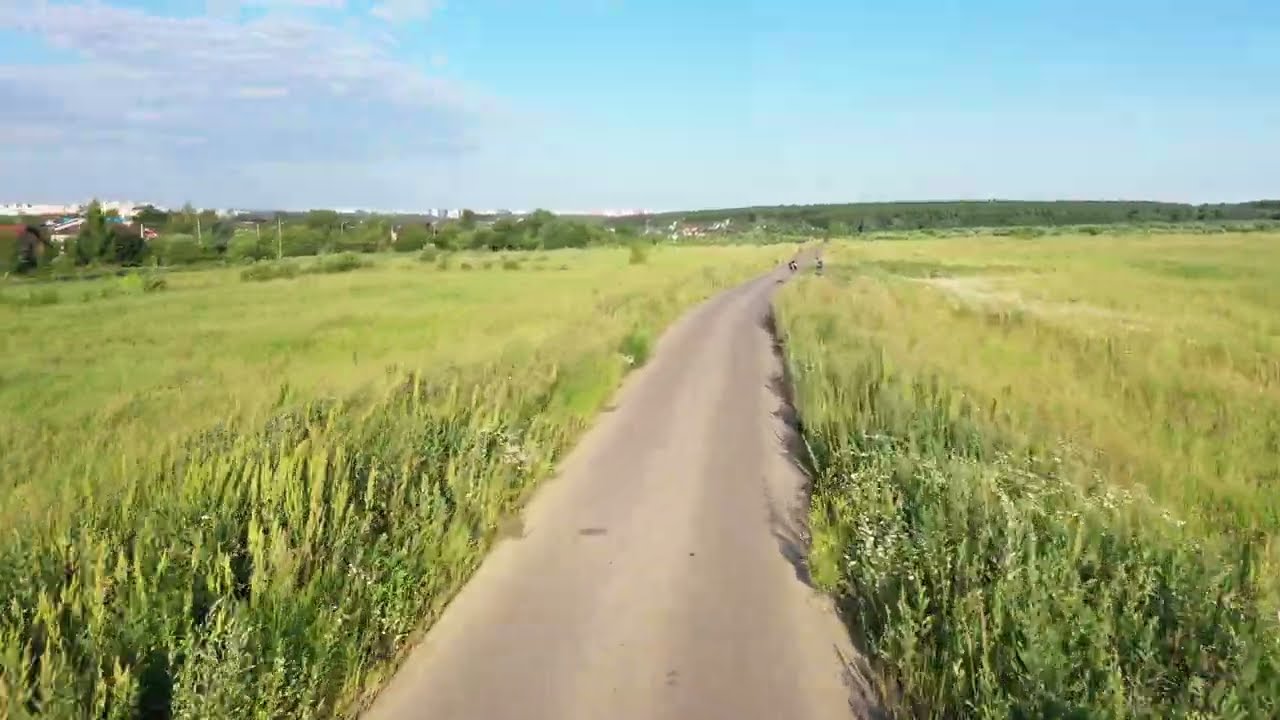The image depicts a small, unmarked dirt road meandering through expansive grassland and farmland. The road, which exhibits two light ruts from tire tracks, stretches into the distance under a clear, partly cloudy sky. Flanked by wild, irregularly growing vegetation and tall grasses, the scene is lush and green. Scattered white flowers dot the meadows beside the road. Far off on the horizon, some buildings and line of trees pepper the landscape, while a small, green hill rises to the right of the image. The few structures present, adorned with some street lights, punctuate the otherwise open, rural expanse.